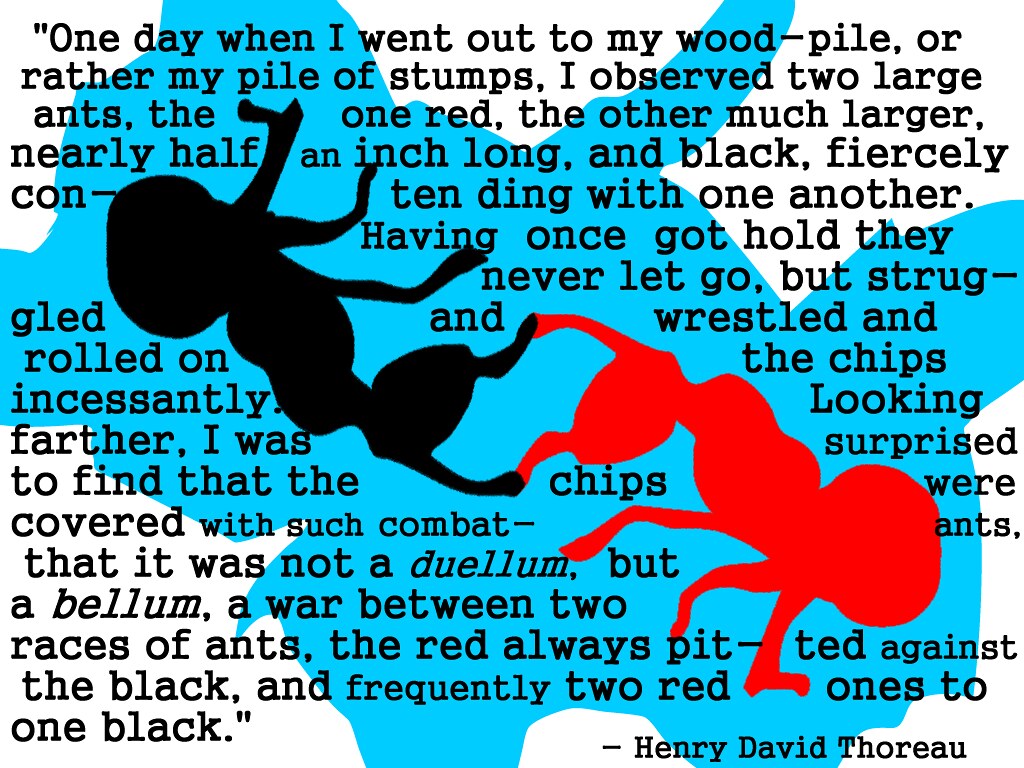The image features an articulate and artistic presentation of a quote by Henry David Thoreau. Set against a white background, the design is highlighted by an abstract, blue splotch that does not cover the entire space. Within this blue blob, two ants—one red and one black—are depicted, appearing almost as if they are engaged in a struggle, with their antennae touching. This creative visualization complements the text of the quote, which is rendered in black letters. The quote reads: "One day when I went out to my woodpile, or rather my pile of stumps, I observed two large ants, one red, the other much larger and black, fiercely contending with one another. Having once got hold, they never let go, but struggled and wrestled and rolled on the chips incessantly. Looking farther, I was surprised to find that the chips were covered with such combat ants that it was not a dwellum, but a bellum, a war between two races of ants, the red always pitted against the black and frequently two red ones to one black." This text captures the essence of Thoreau’s observation of the vigorous, relentless battle between two different races of ants.